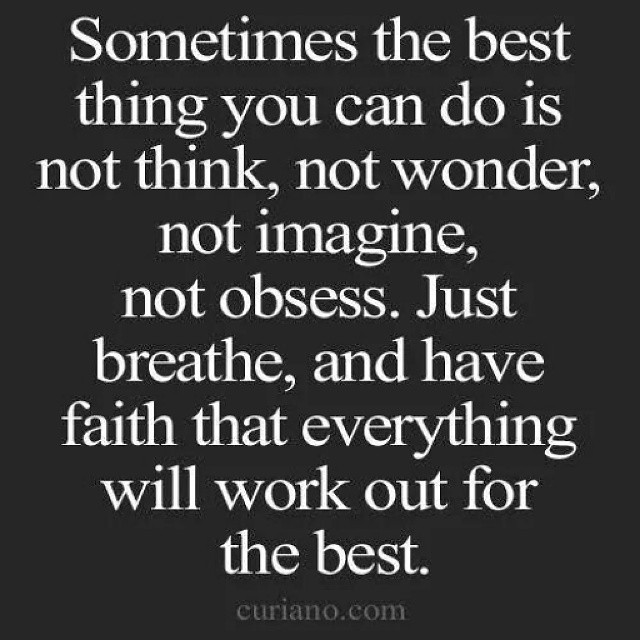The image features an inspirational message in white lettering on a completely black background. The text, spread across nine lines, reads: "Sometimes the best thing you can do is not think, not wonder, not imagine, not obsess. Just breathe, and have faith that everything will work out for the best." Below this uplifting phrase, the website "Curiano.com" is listed in light gray text, subtly different from the main message's bright white. The stark contrast between the black background and the white and gray text makes the motivational message stand out prominently.